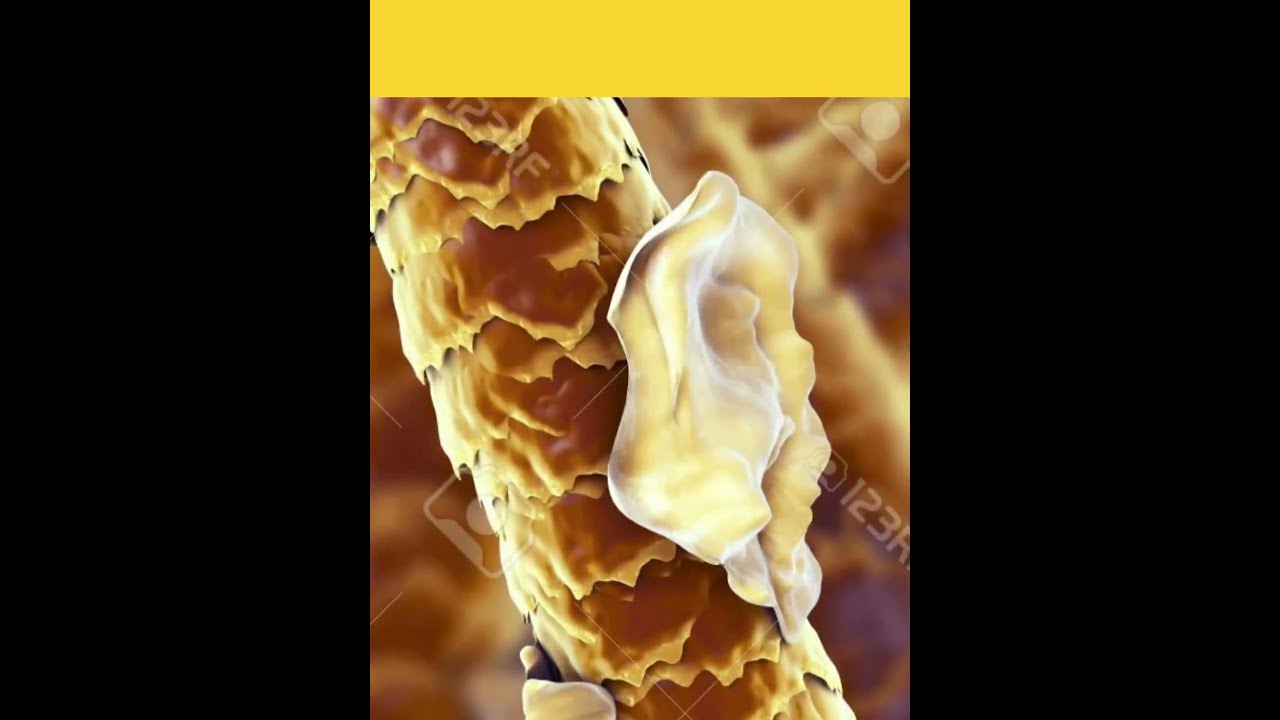This highly detailed microscopic image captures an extreme close-up of a dark brown hair strand with light brown accents. Two thick black strips frame the image on both sides, and a broad yellow band spans the top 10%. The hair is intriguingly ensnared by a white, flat, and wavy fungal growth that somewhat resembles a pig ear in both color and shape. The background reveals additional hair particles, suggesting a magnified, scientific examination. Overlaid on the image are watermarks featuring the text "123K" and "123RF," possibly indicating the original source. A small icon, reminiscent of a camera or a person's silhouette, is centered within the watermark, affirming its digital archival intent.